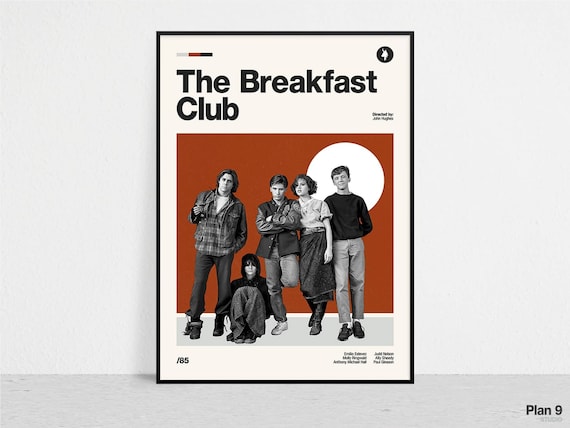The image is a vertically framed movie poster for the classic film "The Breakfast Club," bordered by a thin black frame. Dominating the white background at the top is the film’s title, "The Breakfast Club," in bold black letters. The bottom section of the poster features the five iconic main characters set against a red background. Among them are three men and two women, all initially portrayed in black and white. One of the male characters, distinguishable by his leather jacket, stands next to another man in a varsity jacket, and a nerdy guy with a black sweater and long khaki pants who has a white, globe-like spot or sun behind his head. The most prominent female character, played by Molly Ringwald, is dressed in a dress, standing next to the rebellious goth girl with black hair who is sitting on the floor. In the lower right corner, there is written text that is too small to read clearly, except for "Plan 9." Additionally, in the lower left quadrant, the numbers '85' followed by a forward slash are visible. The overall design suggests it could be a cover for a DVD or book showcasing the memorable ensemble cast of this beloved 1985 film.